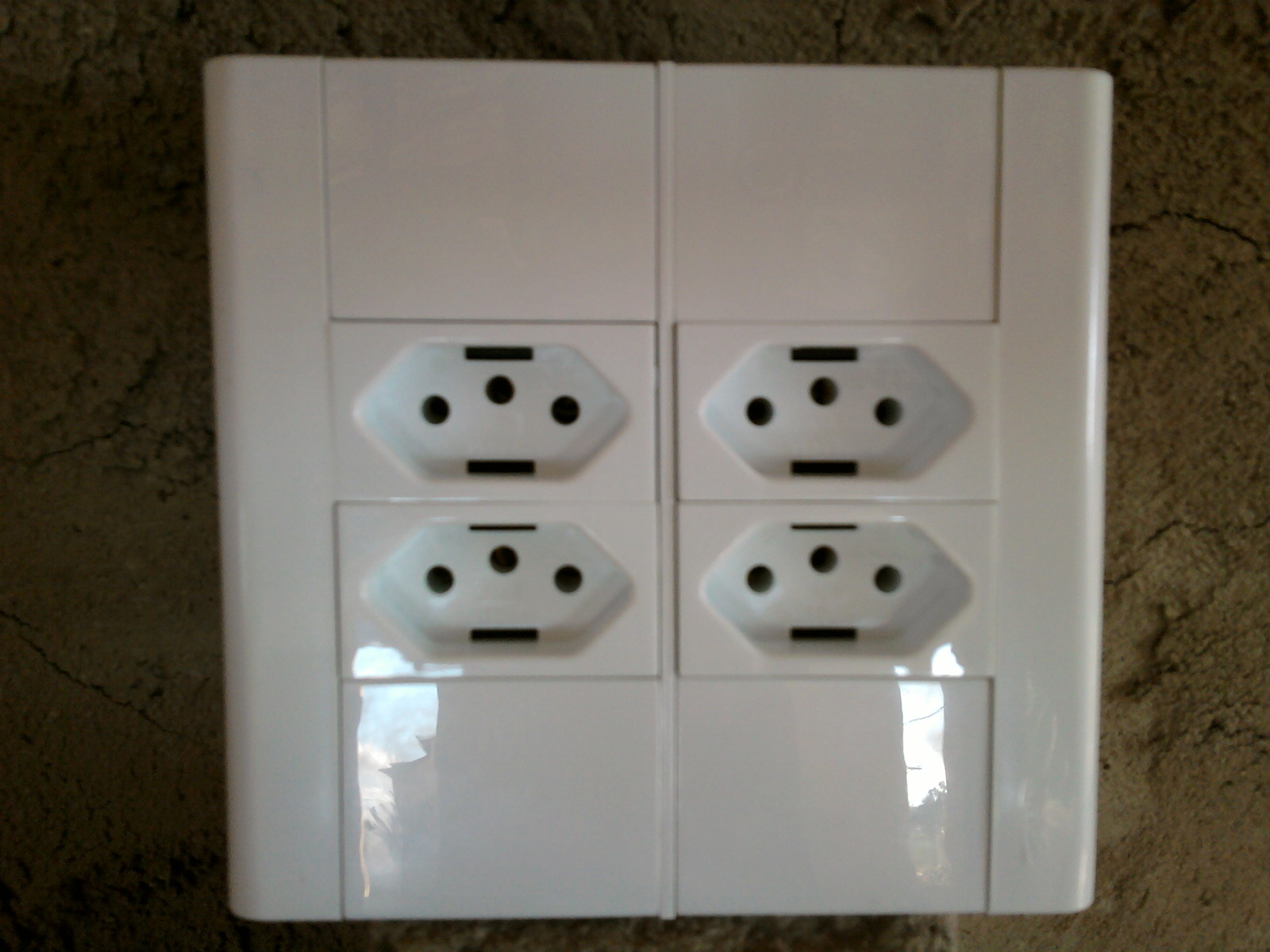The image is a slightly blurry color photograph taken indoors, showing a large, white, glossy plastic square tile. The tile is divided into sections by horizontal and vertical lines, forming a grid pattern. At the center of the tile are four rectangular sections arranged in a 2x2 grid. These rectangles each contain a raised, elongated hexagonal shape. Within these hexagons are two black bars at the top and bottom, and three staggered black circles in a line down the center. The background behind the tile is a rough, brown marbled surface that appears to be granite. The shiny surface of the tile reflects a window with a bright blue sky, some shrubbery, a building, and telephone lines outside, indicating that the photo was taken during daytime.